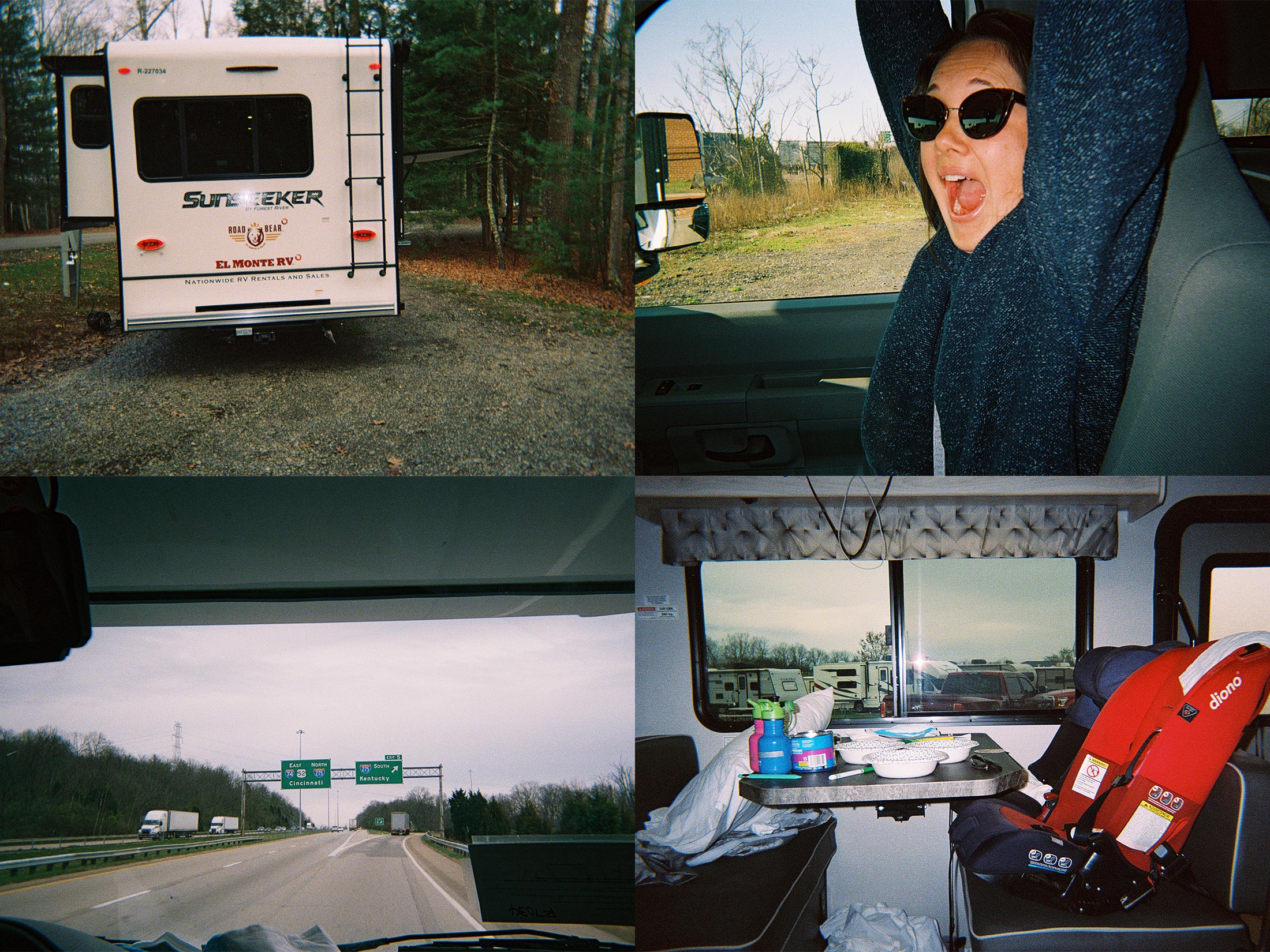This collage of four images, arranged in a grid of two rows and two columns, vividly captures the essence of a road trip in an RV named "Sunseeker." 

In the top left photo, the back of a white RV is seen parked in a driveway, surrounded by trees. The RV features a ladder and an open door, creating a welcoming and adventurous feel. The top right image depicts a Caucasian woman wearing sunglasses and a scarf, seated inside the RV. She has her arms raised and mouth open as if in surprise or excitement. The background through the window reveals a grassy area and a street, indicating a brief stop.

The bottom left image offers a view from the driver’s perspective, showcasing a stretch of Highway 75 South, likely in Kentucky. The RV appears to be in the exit lane, with semi-trucks visible in the opposite lane and highway signs indicating an upcoming exit. 

In the bottom right photo, the inside of the RV is shown in detail. The dining table is cluttered with various items including plates, bowls, cans, and some red car seats to the right, hinting at traveling with kids. Blue and pink water bottles and a white pillow on the left add to the cozy, lived-in atmosphere. Through the window with a small curtain, other RVs can be seen parked outside against a backdrop of greenery.

This series of images collectively captures the dynamic and multifaceted experience of an RV road trip, filled with moments of travel, rest, and the bustling life inside the vehicle.